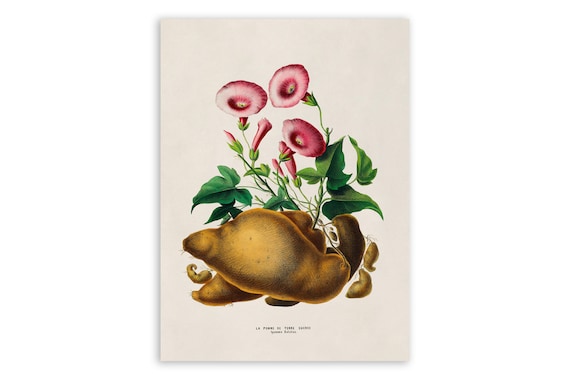This is a detailed botanical illustration set against a pale pink background, depicting a cluster of tubers resembling russet potatoes or yams, with several pointy-ended roots. Emerging from these tubers are lush, dark green, pointy leaves. Rising from the foliage are various stages of blooming flowers, predominantly bright pink and trumpet-shaped. These three large flowers are accompanied by smaller buds and budding flowers, adding depth to the scene. The illustration is colorful and artistically rendered, with a tiny, possibly French, text at the bottom, which remains illegible. The image is vivid and detailed despite being a small photograph.